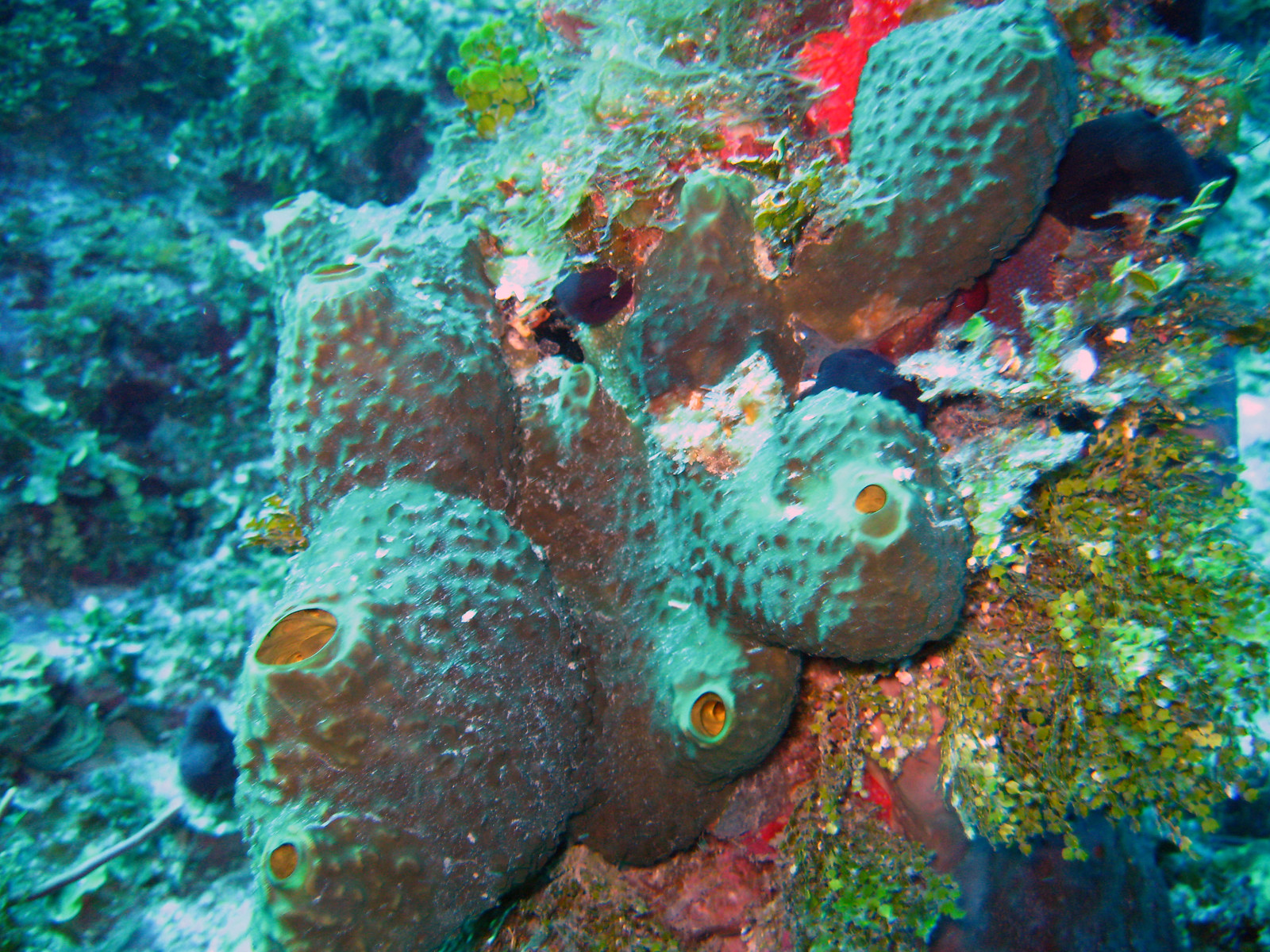This square color photograph depicts a nondescript underwater scene, likely from an aquarium given the surroundings and artificial appearance. The backdrop is dominated by a blend of blue and green hues, rendering a somewhat rocky and crusty environment. The right-hand side continues this theme with similar coloration and texture, accented by additional crusty green and blue bits. 

At the center of the image, several rough-textured lumps resembling sea cucumbers can be seen, each featuring a small opening at the top. These objects are interspersed with pink areas and worn patches that suggest chipped paint, adding to their artificial feel. Further enhancing the aqua illusion, a light turquoise color illuminates the entire scene, suggesting proximity to the water's surface. 

Additionally, there's a piece of coral with a hard surface, adorned with small dots and yellow holes, giving the appearance of glowing from within. Surrounding this coral, one can see some tentatively identified undersea plants: a few grassy strands and small white flowers towards the bottom right, and a dark red area glowing just behind it, the nature of which remains uncertain. 

Overall, the image exudes a sense of undersea tranquility bathed in blue-green light, complemented by assorted marine elements in varied states of realism and color.